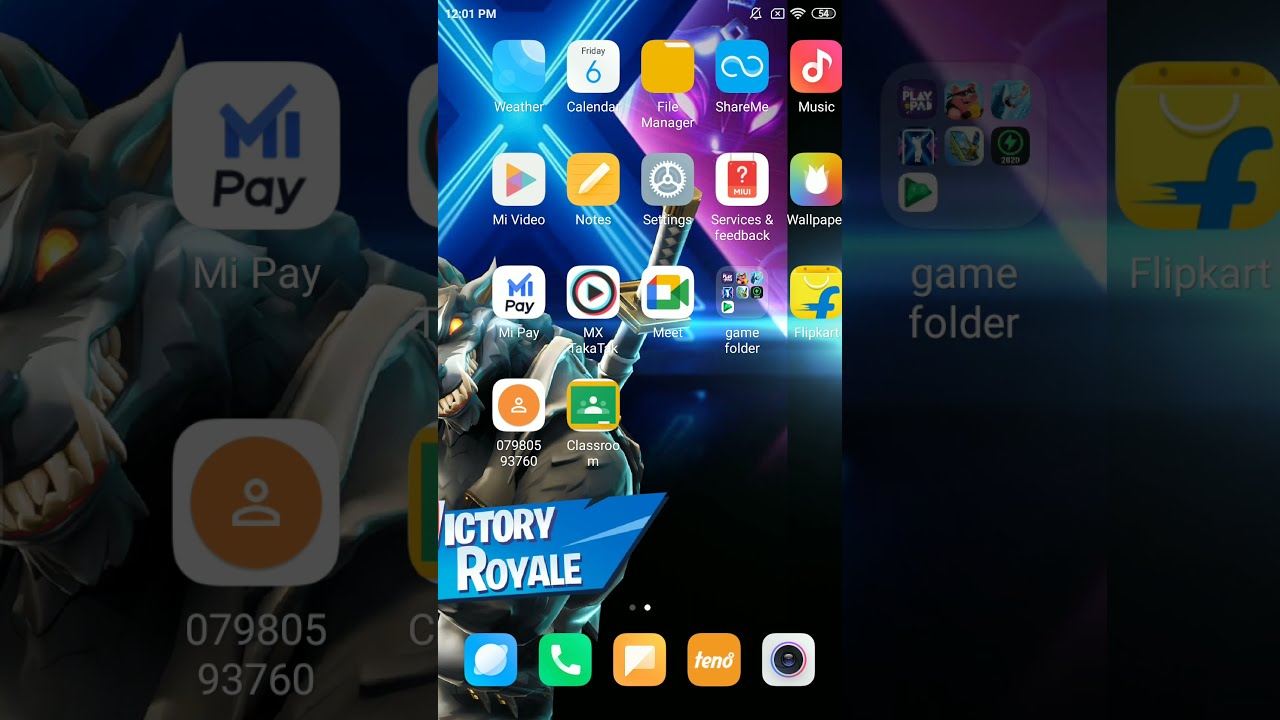The screenshot displays the screen of a smartphone, divided into three sections with the central section being the brightest and the left and right sections heavily tinted. The central section showcases a grid of numerous app icons placed in rows from top to bottom. The first row consists of icons for Weather, Calendar, and File Manager. The second row includes Share Me, Music, My Video, Notes, Settings, Services and Feedback, and Wallpaper. Following that is a row featuring My Pay, MX, Meet, Game Folder, and a file app labeled File Point. 

An additional row presents two more app icons: one with numerical labels "079805" and "93760," and the Classroom icon next to it. Below these apps is a blue backdrop with the text "Victory Royale" displayed prominently. Adjacent to the "Victory Royale" text are various icons: a blue icon with a planet and an orbiter, a green icon with a phone, an orange icon with a white square, another orange icon labeled "Tint," and a white square symbol that appears to be for taking a picture.

The tinted sections on the left and right sides seem to be zoomed-in portions of the central screen, highlighting specific icons. The left side features a close-up of the My Pay icon and another icon characterized by a yellow circle with an illustration resembling a person's face and shoulders. The right side shows a zoomed-in view of the Game Folder icon alongside the Flipkart folder.

In the background, a menacing monster with bright orange eyes, gray skin, sharp teeth, and a horn on its head stands menacingly. Behind this, a neon X-shaped light further accentuates the dramatic effect of the monster's presence.